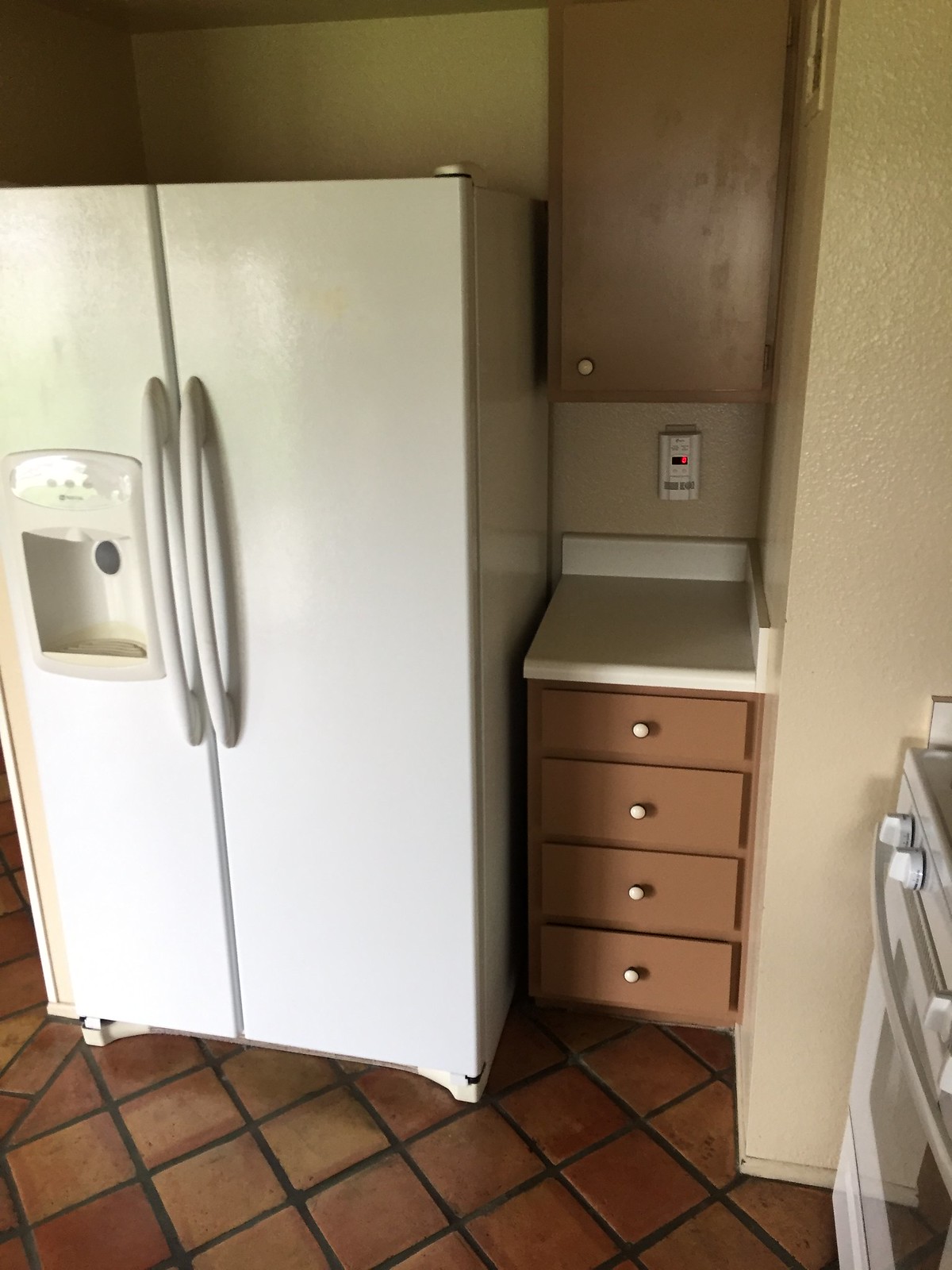This portrait-oriented photograph captures a vintage, snug kitchen interior with a cozy feel. The kitchen features a beige or mustard-colored wall, contrasted by rich brown cabinetry equipped with small white circular knobs. Below the cabinet, a compact counter with four drawers, these being brown with white round handles, sits next to a dual-door, white refrigerator that fits neatly into its space. The refrigerator is equipped with an ice maker and has a section for dispensing water, ice, or crushed ice via three front buttons. The kitchen floor is adorned with red, brown, and copper Mexican-style tiles, outlined with black grout. Adjacent to the refrigerator stands a white stove with four knobs and a slightly curved oven door, hinting at a classic range top. Overall, the coordinated elements and vintage touch give this small kitchen a timeless and charming ambiance.